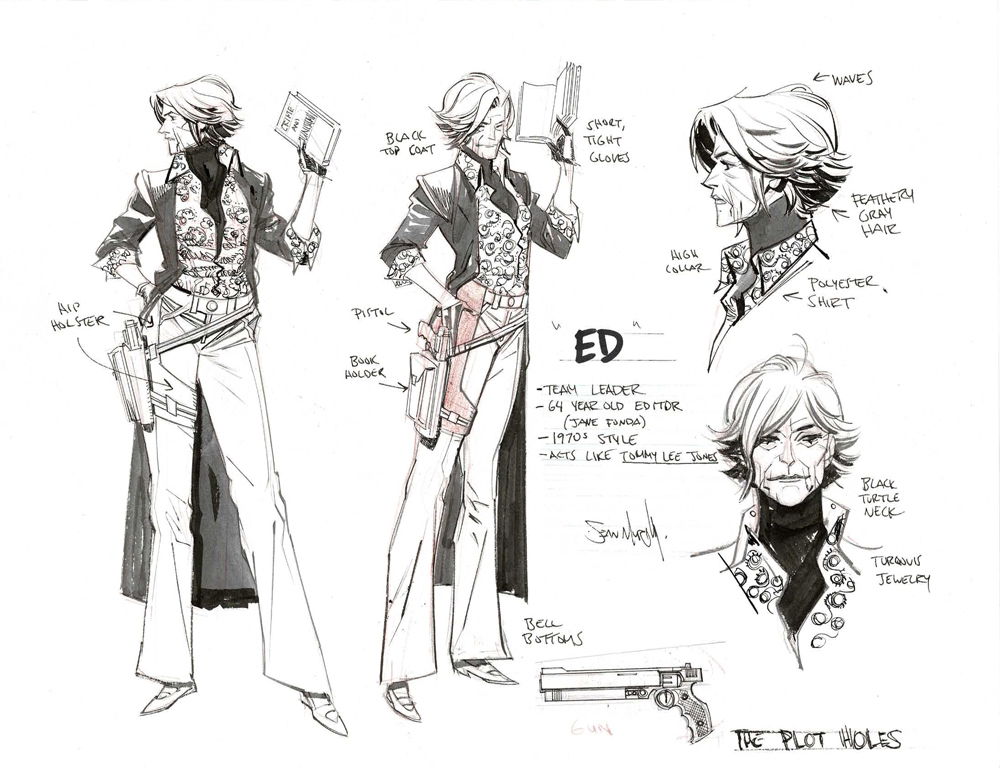The image is a detailed sketch of a character named Edie, a 64-year-old editor, styled after Jane Fonda in the 1970s and with a personality akin to Tommy Lee Jones. The composite sketch features multiple angles and close-up views of Edie, emphasizing her attire and accessories. 

The leftmost image portrays Edie in a full-body pose, with short hair, a long dark duster over a black bolero jacket, and a fancy swirled polyester shirt with patches of pink. She wears light-colored bell-bottom pants, a gun holster strapped to her waist and right leg, and holds a book in one hand, her other arm resting on her hip. Her belt and hip holster are marked in red.

Another depiction shows her at a different angle with an open book held near her face, this time with labels pointing out elements of her outfit and accessories. The descriptions note her black turtleneck, short tight gloves, and prominent, feathery gray hair. Her shirt is high-collared, and she wears bell bottoms.

In the profile view on the right, detailed arrows point to her wavy short hair, lower feathery locks, and high-collared shirt. A head-on sketch highlights her black turtleneck and some type of jewelry. 

Throughout the sketch, detailed notes are added, including descriptors like "waves," "polyester shirt," "pistol," and "book holder." At the bottom right, there is an illustration of Edie's gun, labeled "the plot holes." Overall, the image serves as a comprehensive character design for Edie, showcasing various aspects of her appearance and equipment.